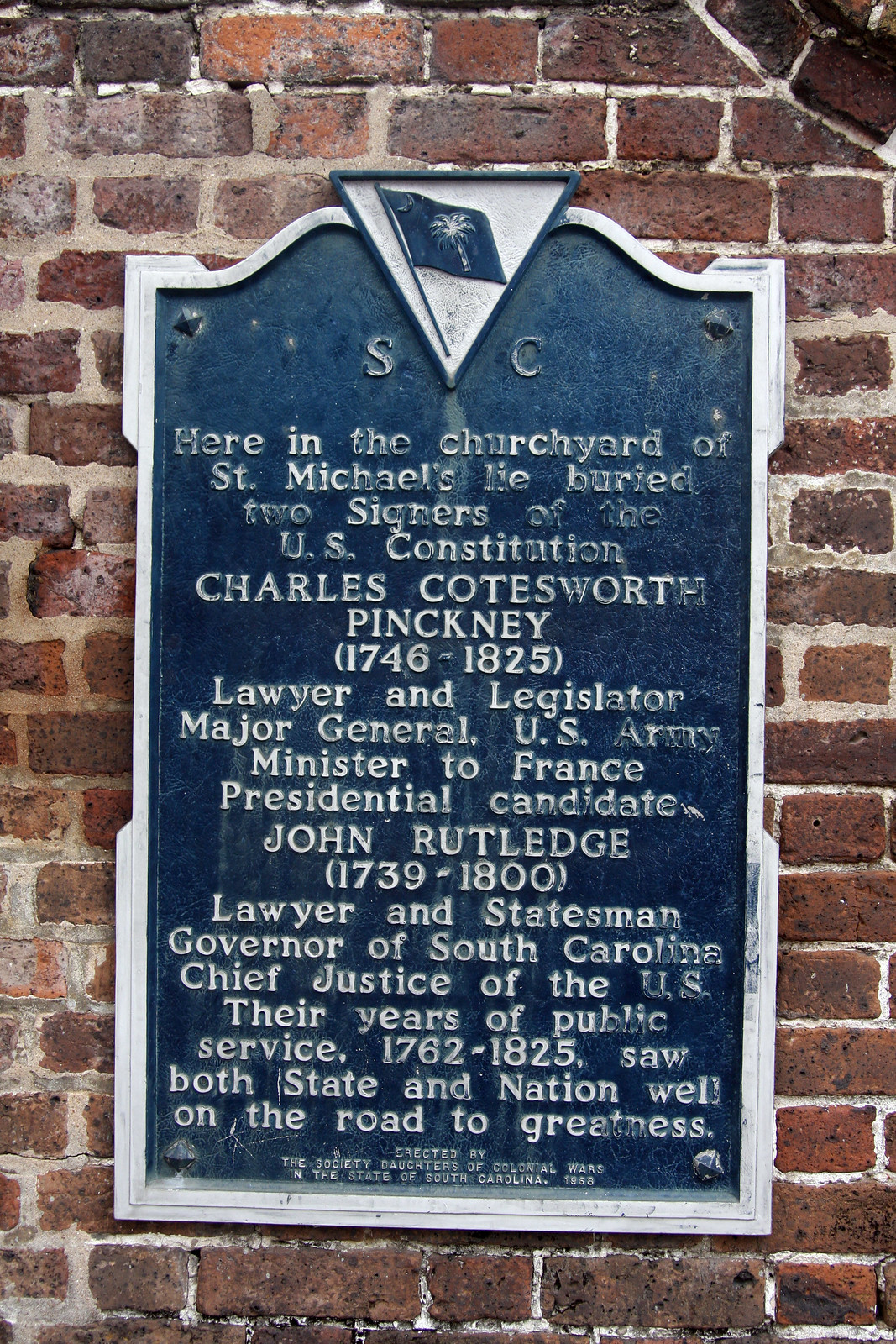The image displays a large, old, and weathered metal plaque bolted to an orange brick wall with white grout. The plaque, framed by a fading blue color with a white border, prominently features the letters "S" and "C" at the top. Between these letters, a navy blue or black drawing of the South Carolina flag with a palm tree and in an upside-down triangle is displayed. Below the flag, in white font, the text reads: 

"Here in the churchyard of St. Michael's lie buried two signers of the US Constitution:

Charles Coatesworth Pinckney (1746-1825)
- Lawyer and legislator
- Major General, U.S. Army
- Minister to France
- Presidential Candidate

John Rutledge (1739-1800)
- Lawyer and statesman
- Governor of South Carolina
- Chief Justice of the U.S.

Their years of public service (1762-1825) saw both state and nation well on the road to greatness."

At the bottom, in small print, it states: "Erected by the Society Daughters of Colonial Wars in the state of South Carolina, 1888." The plaque's appearance is notably aged, with rust and significant color loss, once predominantly blue but now showing signs of wear and time.